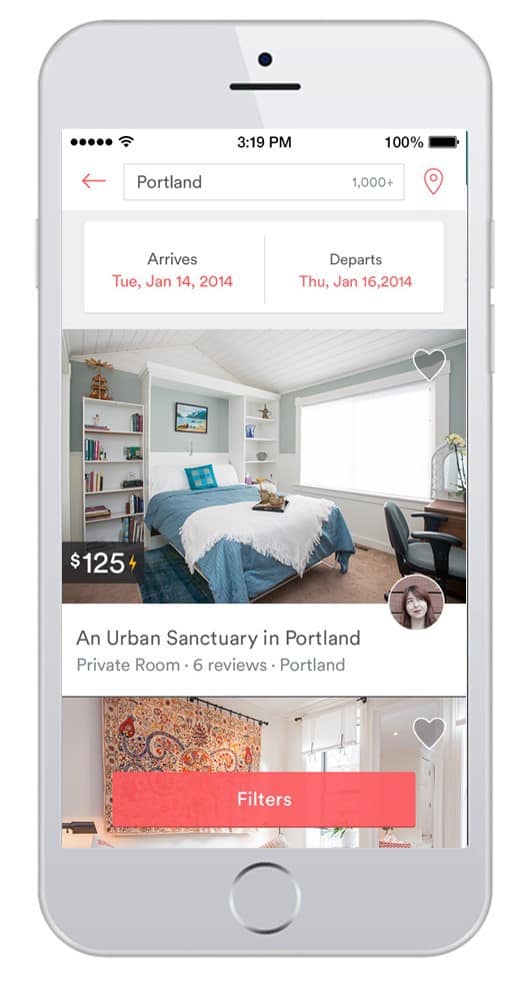The image depicts a screenshot from a mobile phone at 3:19 p.m. with a fully charged battery. It features a detailed advertisement for a room rental in Portland. A prominent red arrow points to the left, and a large search bar contains the text "Portland."

The rental details are specified: arrival on Tuesday, January 14, 2014, and departure on Thursday, January 16, 2014. The image includes a cozy bedroom scene with a neatly made bed adorned with a white and blue blanket. Behind the bed, there are bookshelves filled with books and a compact computer desk.

The cost for the rental is indicated as $125. A profile picture of a woman in a circle is shown, accompanied by the description, "An urban sanctuary in Portland. Private room, six reviews." Below this section, the word "filters" appears. This advertisement serves as a potential invitation to book a stay in this well-appointed bedroom, ideal for someone seeking a comfortable and private accommodation in Portland.